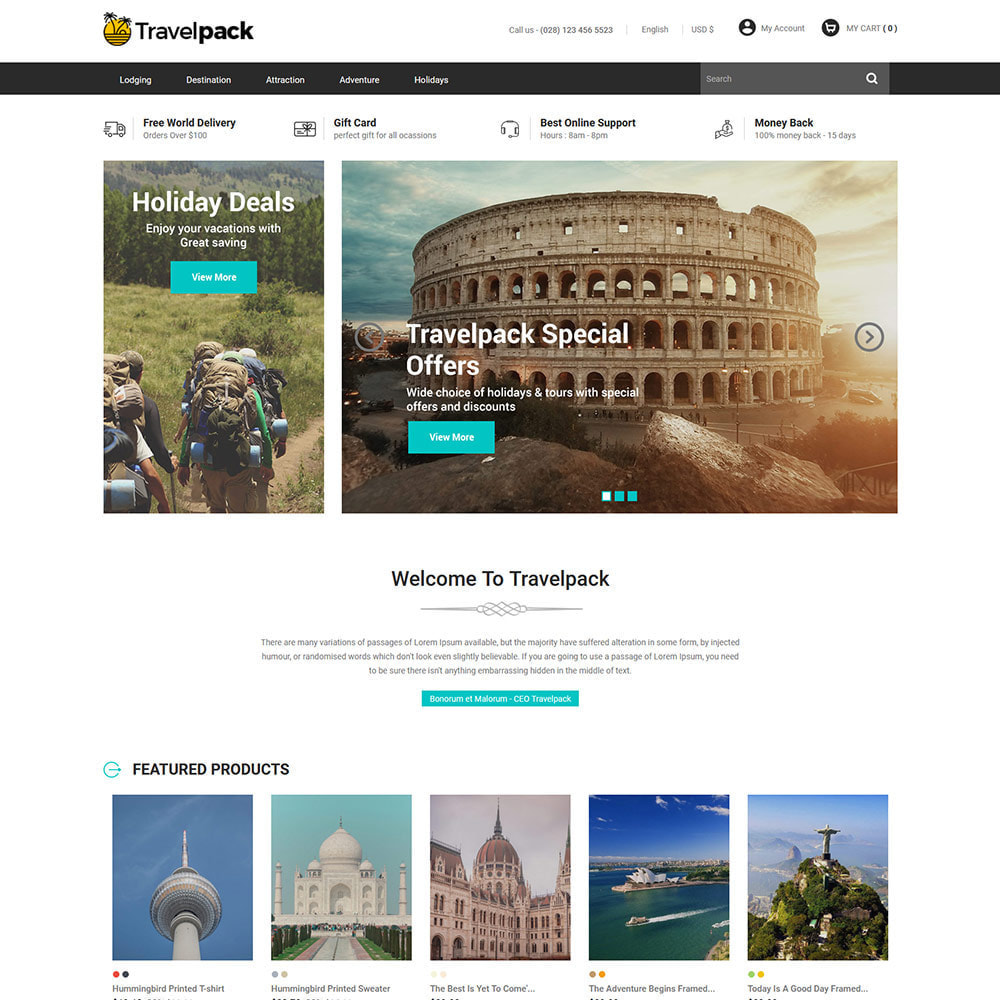The image depicts the landing page of a travel website named TravelPak. The header, which is white, features the TravelPak name on the upper left-hand corner, accompanied by a small yellow logo depicting two palm trees. Directly below the header is a menu strip, with categories that are too small to read clearly. Positioned towards the right-hand side of this menu strip is a search box. 

The main featured area showcases holiday deals, prominently displaying a clickable button labeled "View Here." Over a vivid background image of the Coliseum in Rome, the text "TravelPak Special Offers" is emblazoned in white. Further down, the page welcomes visitors with a "Welcome to TravelPak" message. Subsequent to this, there are featured products section with five photographs spotlighting various travel destinations. The remaining background of the page is predominantly white, maintaining a clean and simple aesthetic.